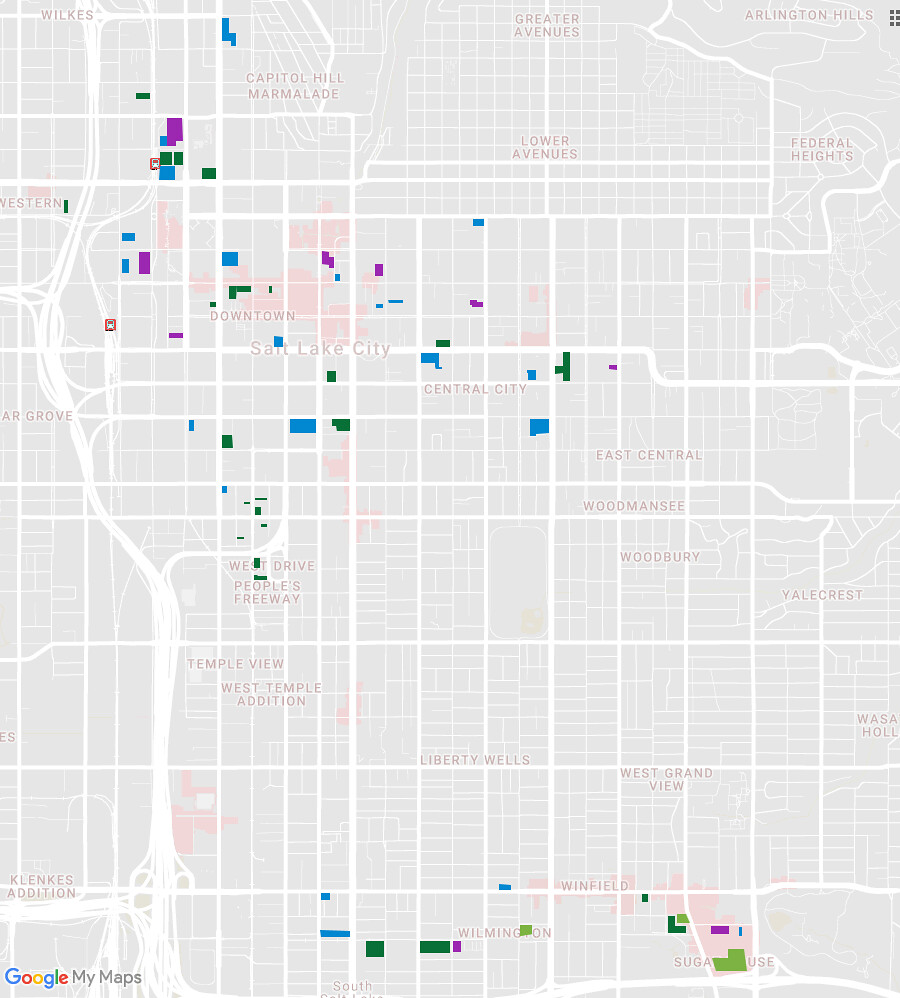This screen capture from Google My Maps visually represents the meticulously planned grid-lined streets of Salt Lake City. The map features a grey background with streets delineated in white, showcasing the city's organized layout. Labels for various neighborhoods and districts, such as Capitol Hill Marmalade, The Western, The Grove, and downtown Salt Lake City, are written in a pale pink color, providing clear distinctions of different areas. Notably highlighted are significant thoroughfares like the West Drive People's Highway, as well as specific locales such as Temple View, West Temple Addition, and Klinkies Addition.

In the lower portion of the image and ascending along the right-hand side, more neighborhoods are identified, including Sugar House, Wilmington, Winfield, West Grand View, Yalecrest, East Central, and Federal Heights, among others. The map is interspersed with small blue, green, and purple rectangles, likely indicating buildings of importance or landmarks. There are also larger pale pink blocks that seem to denote prominent structures or significant building complexes, offering a detailed and vibrant representation of Salt Lake City's urban geography.